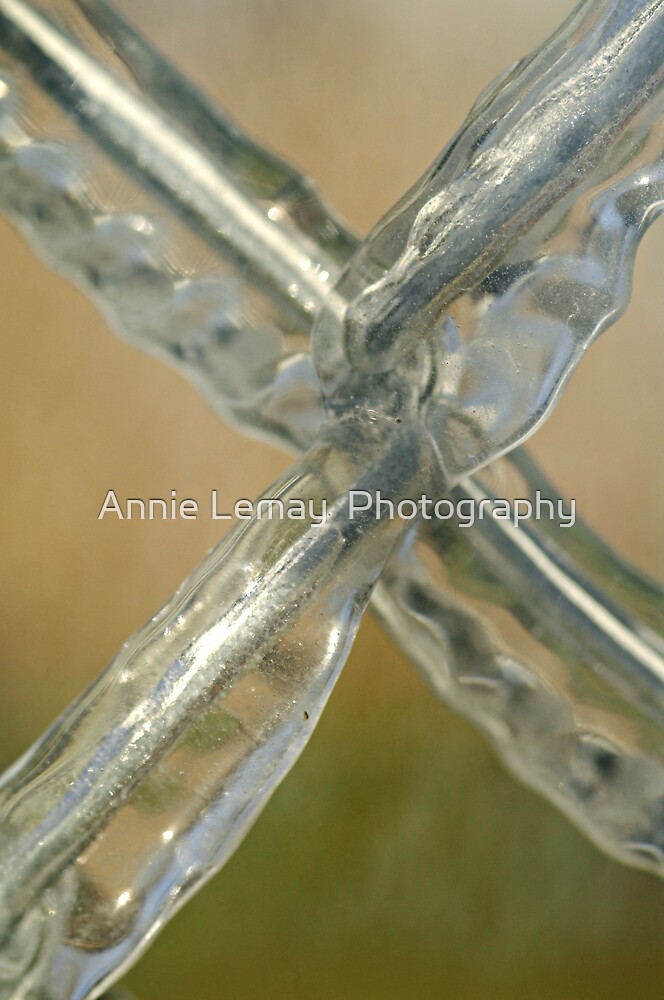The photograph captures an artistic rendering of four silver metal pieces intersecting centrally, resembling a chain-link fence covered in a substance that appears to be ice. The metallic elements cross to form an 'X' shape, creating an intricate, icy latticework. The backdrop features a faded tan color transitioning to green at the bottom, suggesting grass. At the center of the image is a small overlay text, reading "Annie LeMay Photography" in a modern white font with a black shadow, adding a professional watermark to the composition.